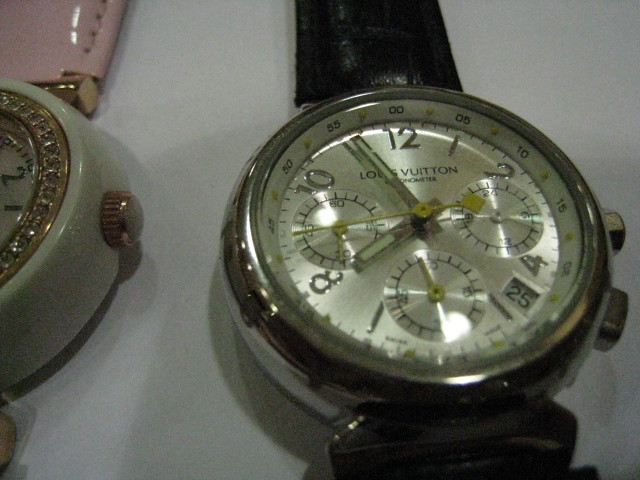This close-up photograph captures two wristwatches lying on a gray background. The watch on the right, likely a man's watch, features a black leather band and a chrome metal casing with a silver metallic face. It prominently displays the Louis Vuitton logo in gold against its silver center. The watch face includes silver numbers from 12 to 11, with lines marking seconds, three additional dials for unknown functions, and a date display set to the 24th. The hour and minute hands are silver with white centers, indicating a time of approximately 7:56, while the yellow seconds hand points to 55 seconds.

To the left, there is a woman's watch with a bubblegum pink leather band. Its white base is trimmed in gold, and the rim around the face is adorned with a single row of what appear to be small diamonds. This watch also has a gold-colored dial on the side. Although only partially visible, the watch face is white with black numbers, and the number 2 is discernible. The overall image has a subdued lighting, suggesting it may have been taken in dim conditions.